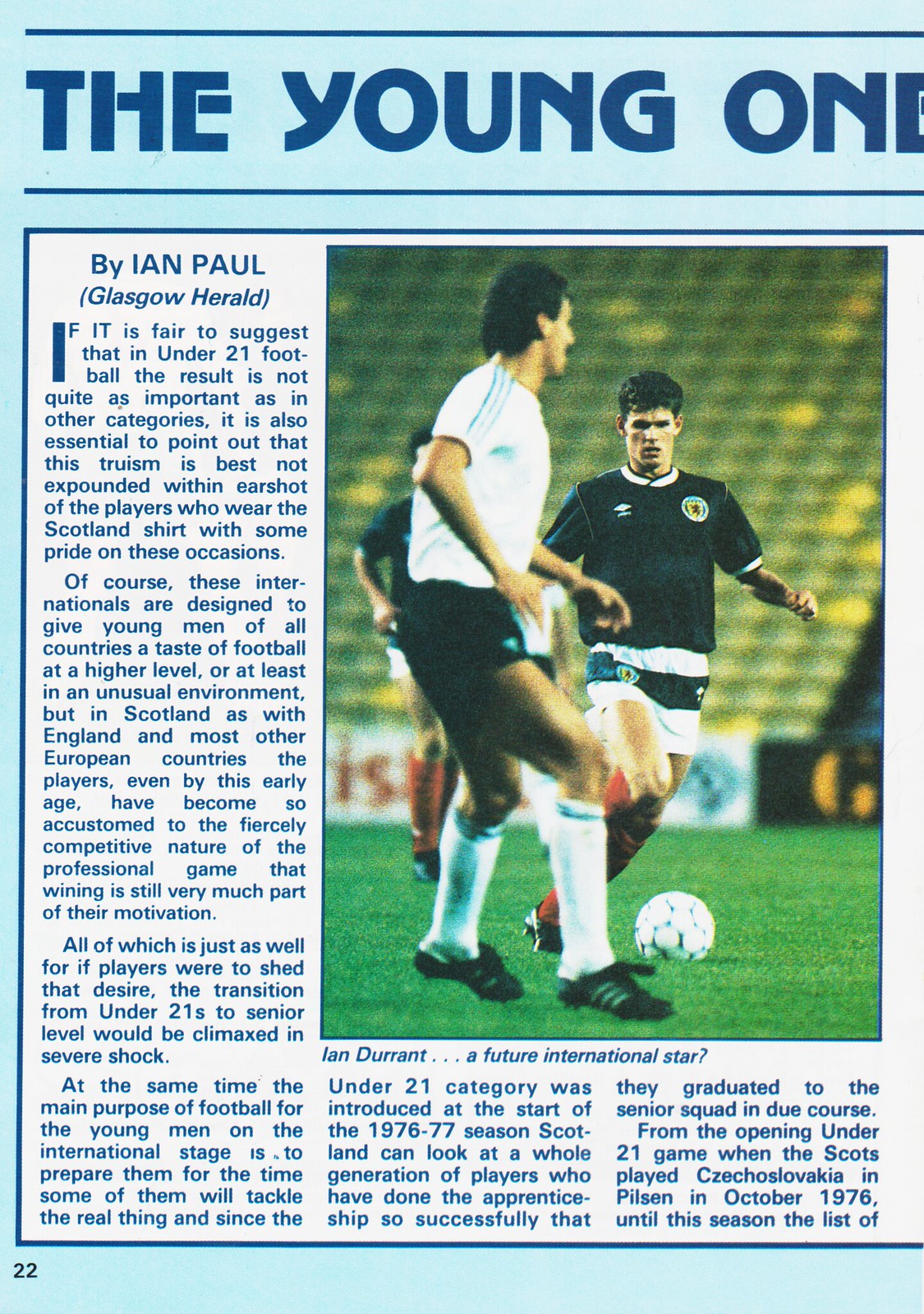This image appears to be a clipping from a book, magazine, or newspaper article. The image features a large photograph on the right side, showing three soccer players on a grassy field, all wearing black and white jerseys with red socks. One player is about to kick a white soccer ball. A game official, dressed in a white shirt, white socks, and black shoes, stands in the foreground. In the background, stands filled with spectators are visible. The photograph is captioned "Ian Durant, a future international star?" 

On the left side and bottom of the image, there is text. At the top, it says "The Young One" in bold blue font on a light sky blue background. The article is by Ian Paul from the Glasgow Herald. The first paragraph reads: "If it is fair to suggest that in under 21 football, the result is not quite as important as in other categories, it is also essential to point out that this truism is best not expounded within earshot of the players who wear the Scotland shirt with some pride on these occasions." The article continues across several paragraphs, featuring multiple colors of text including white, light blue, dark blue, black, green, yellow, tan, and a little bit of gray.